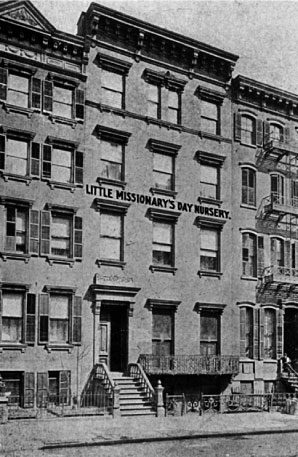This black-and-white photograph captures a tall, four-story building that prominently displays a sign reading "Little Missionaries Day Nursery" across its midsection. The structure features two windows per level on the left and three per level in the middle section, indicating the presence of multiple rooms or dormitories. An open, somewhat dark front door is accessed by a set of elaborate, curved steps flanked by decorative pillars. To the right, railings for each level are visible, likely part of fire escapes, further emphasizing the building's aged character. The bottom part of the building features wrought iron gates, hinting at a gated section. The scene is devoid of cars and trees, focusing solely on the striking building against a gray, grainy sky, with a road and sidewalk lying in the foreground.